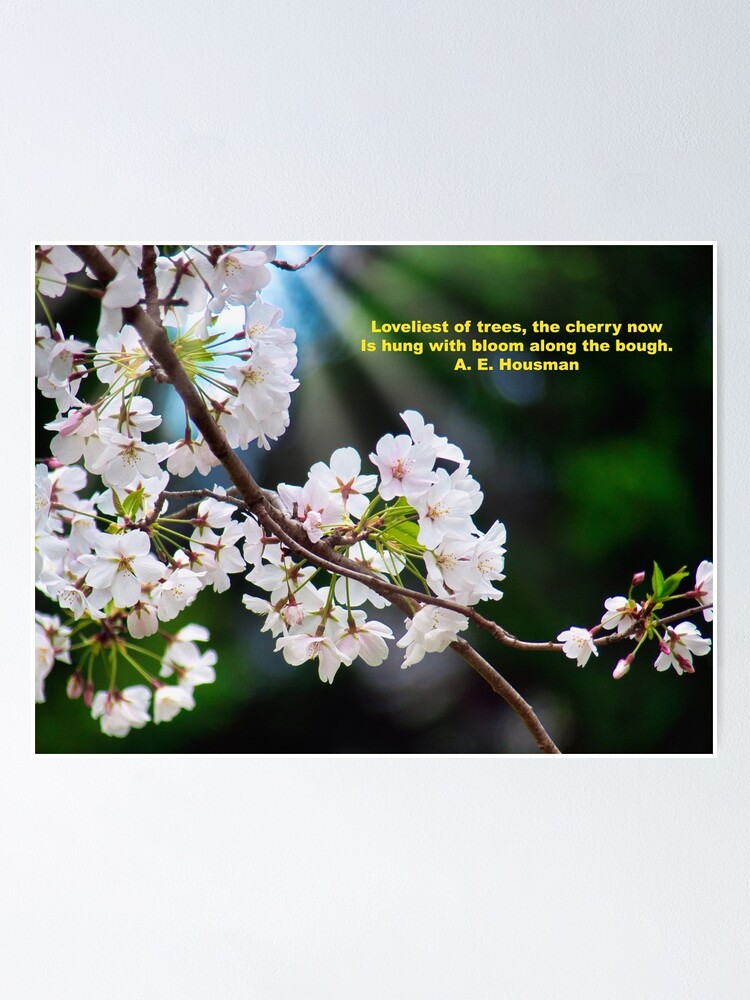The image showcases a photorealistic depiction of a cherry blossom tree branch, extending diagonally from the top left to the bottom right. The branch is adorned with clusters of cherry blossoms, displaying delicate white petals with pink centers. Alongside these blossoms, there are smaller green flowers observed below the white ones. The branch bifurcates near the middle, with a smaller offshoot extending to the right, also featuring a blossoming flower at its tip. The left third of the image is dense with these striking cherry blossoms, adding a sense of flourishing nature. The background is blurred, featuring splotches of green and gray with a sunny glow, suggesting a sunlit day. In the top right corner, in yellow text, is the quote: "Loveliest of trees, the cherry now is hung with bloom along the bough," followed by "A.E. Housman." This textual addition lends an evocative poetic touch to the serene and beautiful scene.